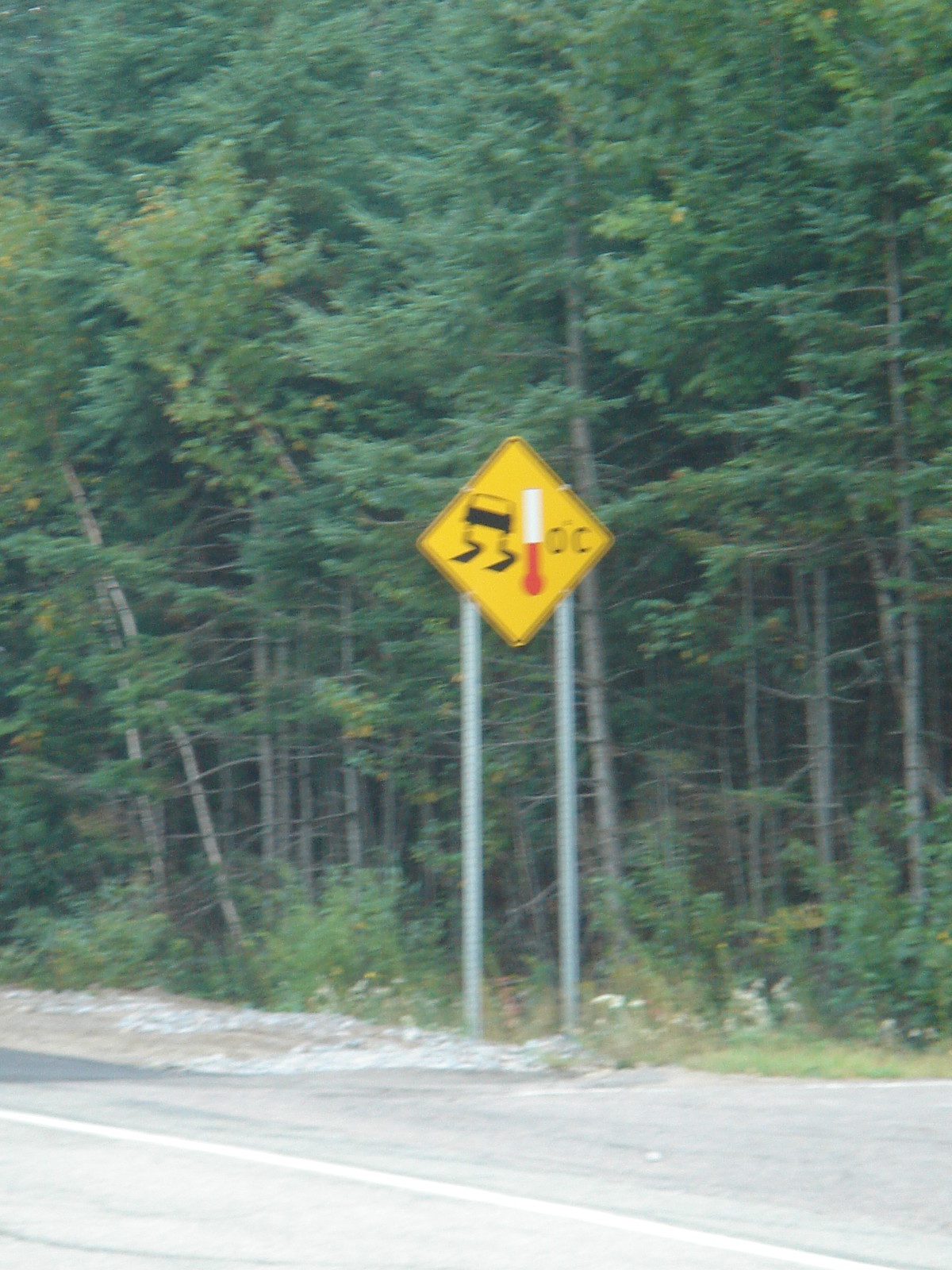In this outdoor photo, a forest with dense green trees forms the backdrop. Positioned on the roadside, there's a yellow diamond-shaped sign supported by two metal poles. The sign features an image of a black car skidding with wavy lines trailing from its rear wheels, indicating slippery conditions. To the right of the car image, there’s a thermometer that’s half red and half white, displaying "0°C" next to it. Surrounding the sign at the bottom are asphalt and scattered rocks. A solid white line runs through the middle of the road. The image captures the scene from across the street, emphasizing the thick forest and the road’s shoulder.